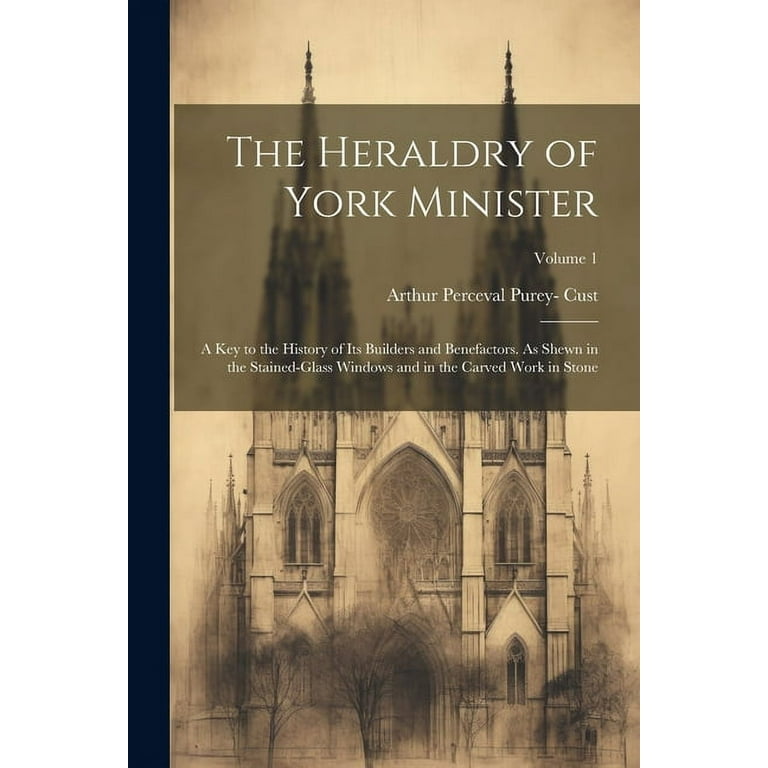The image is the cover of a book titled "The Heraldry of York Minster, Volume 1" by Arthur Percival Percy Cust. The background features a detailed pencil drawing of an old cathedral with two tall spires flanking the symmetrical façade, which includes an arched door and arched windows. Leafless trees stand in the foreground, contributing to a somewhat somber, dreary mood. The cover has a vertically aligned rectangular design, with a vertical black border on the left side and a brownish hue overall. Towards the top, against a darker brown background, the title and subtitle are arranged in right-aligned, all-caps white text. Beneath the main title, it reads "Volume 1," followed by the author's name, and further down, the subtitle: "A key to the history of its builders and benefactors as shown in the stained glass windows and in the carved work in stone." The cover also has some dark brown stains near the bottom, where the sketch includes trees.